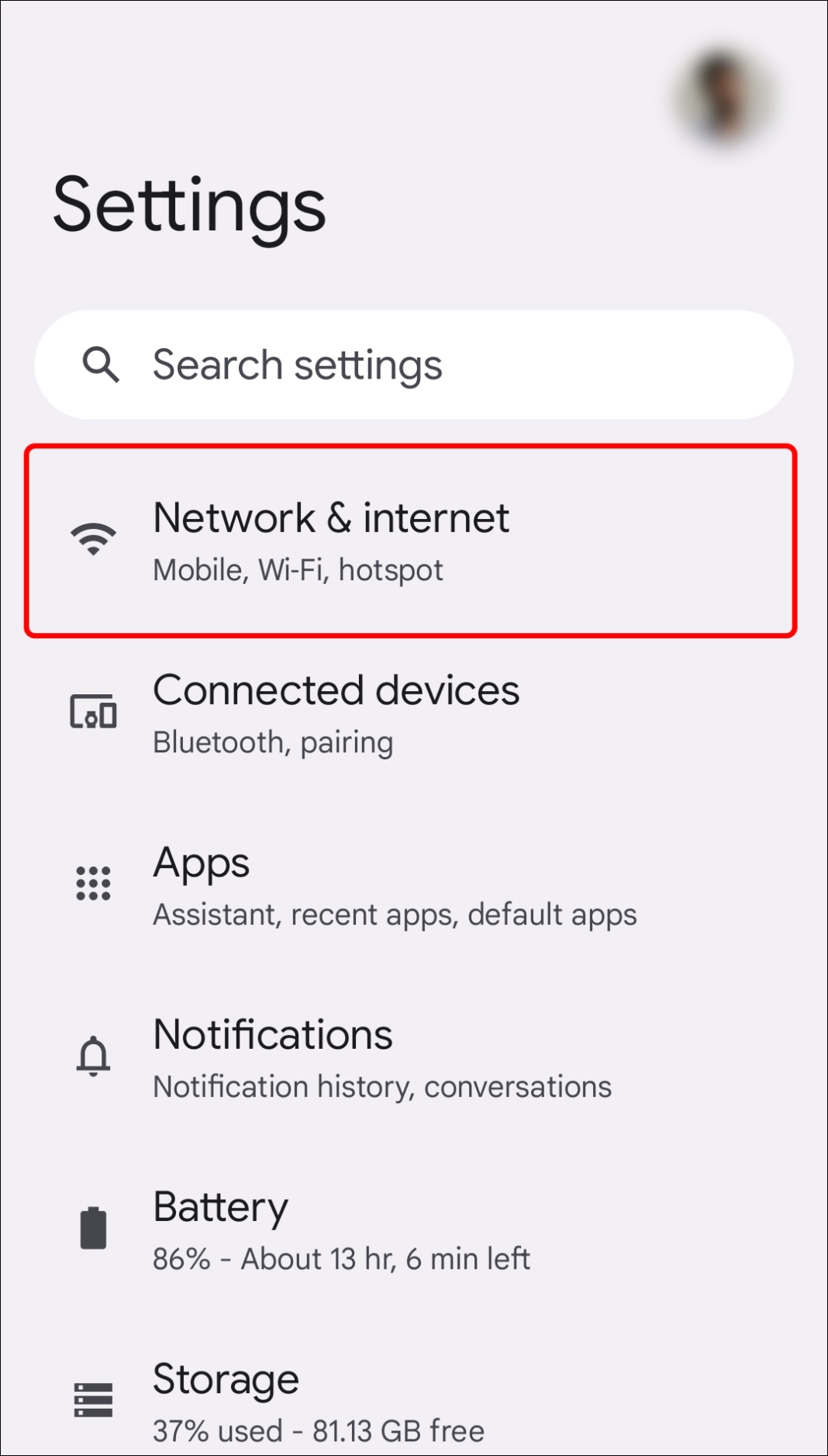This image depicts a vertically oriented screenshot of the Settings section from an Android phone's interface. The background is predominantly gray, and in the upper right corner, there appears to be a slightly blurred circular black image, likely representing the user's avatar. 

On the left side, there is a bold black "Settings" label. Directly below it, a large white search bar is present, identified by a gray magnifying glass icon and the text "Search settings."

The first outlined section is a red-bordered button featuring a Wi-Fi symbol on the left and labeled "Network & internet." Below this, there is a subtitle that reads "Mobile Wi-Fi hotspot." 

Following this, there is a series of settings items without outlined boxes:

1. An icon resembling a monitor/phone on the left, labeled "Connected devices." Underneath, in lighter text, is "Bluetooth, pairing."
2. An icon with three rows of three black dots forming a square, labeled "Apps." Below this, in gray text, are the words "Assistant, recent apps, default apps."
3. A bell icon next to the label "Notifications." Underneath, in lighter text, it reads "Notification history, conversations."
4. A fully charged battery icon to the left of the label "Battery." Below this, in fainter text, it states "86% - about 13 hr, 6 min left."
5. An icon showing three horizontal gray bars with a white dot on each, labeled "Storage." Below this, in light gray text, it notes "37% used - 81.13 GB free."

This detailed caption accurately describes the settings section on an Android phone, not an iPhone as initially suggested.